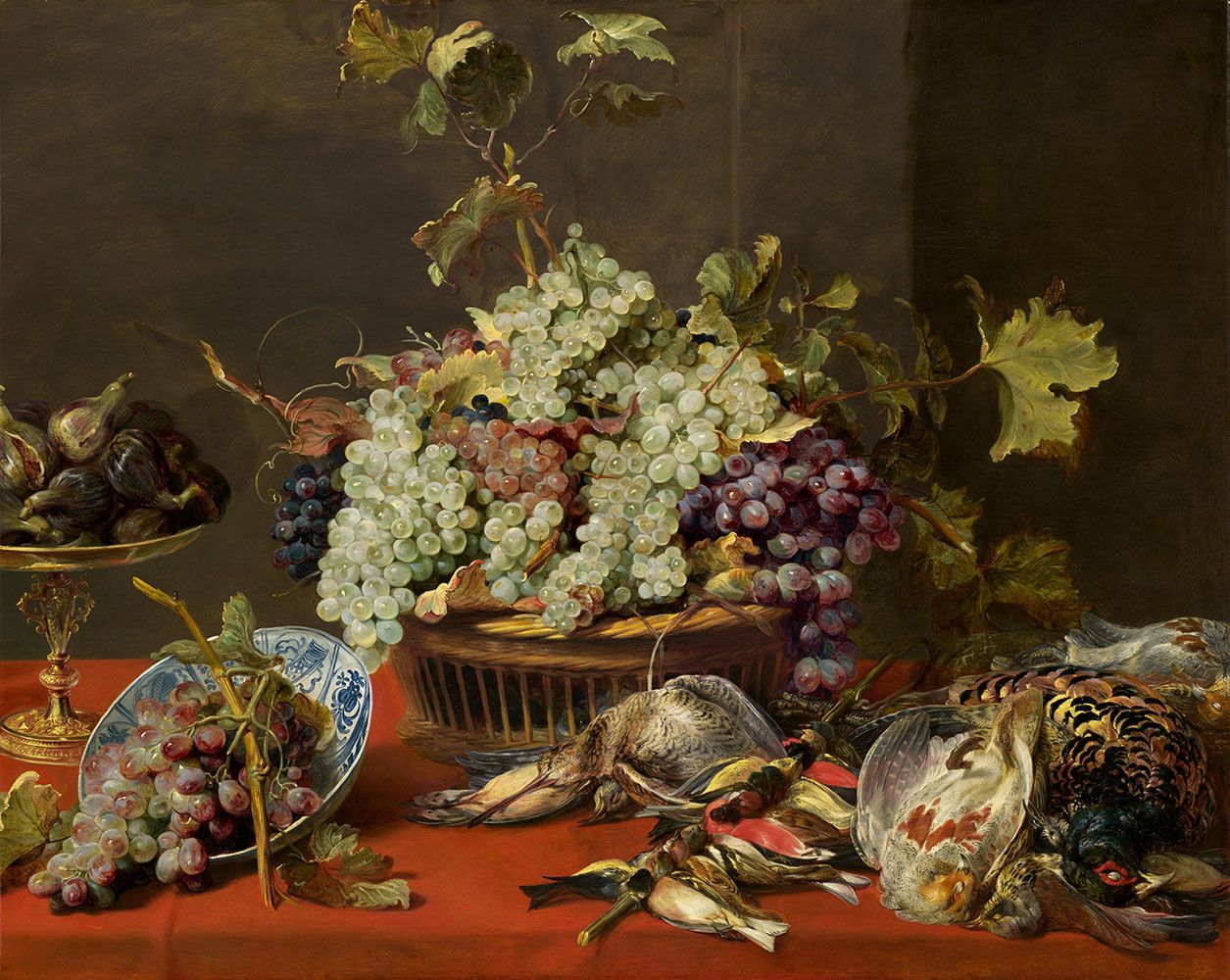The image depicts a hyper-realistic painting in what appears to be acrylic or oil-based medium. The scene is set on a long table draped with a red patterned tablecloth. At the center of the table, there is a large, intricately woven brown wicker basket filled with a heaping mass of grapes in varying shades of green, purple, and black, accompanied by lush green leaves. To the bottom left, a fine china bowl, blue and white in color, holds a smaller bushel of purple and green grapes, complete with leaves and a large brown stem. Adjacent to the basket, a golden, ornate platform dish displays a selection of fruits, likely dates or figs, in dark brown and light green hues. Scattered in front of the basket are several dead birds, intricately detailed with vibrant feathers in red, gold, brown, white, and black. These birds are stacked on top of each other on the right side of the table, contributing to the ambiance of a Victorian-era still life feast.